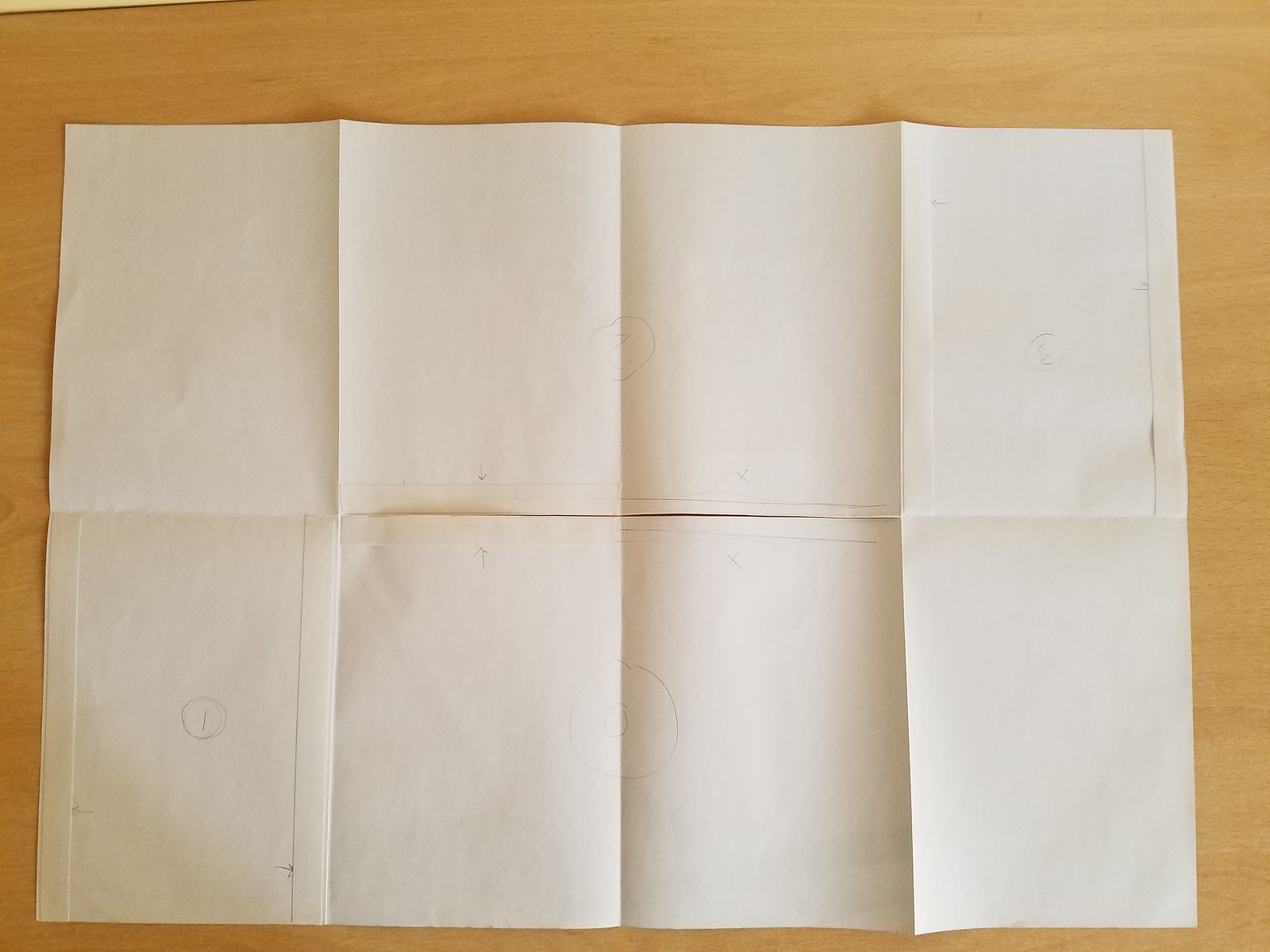A photograph captures a sheet of paper resting on a beige wooden surface, with a small portion of the wood's edge visible in the upper right corner. The paper appears to have been folded eight times, positioned so that its longest side aligns horizontally and its shortest side vertically. Notably, there is a vertical cut in the middle of the sheet, removing a significant portion from the center. The paper bears faint, lightly penciled doodles, featuring a mix of circular shapes and numbers, encased within circles. These numbers range from 0 to 3, with the 1 and 0 located in the lower half and the 2 and 3 in the upper half.